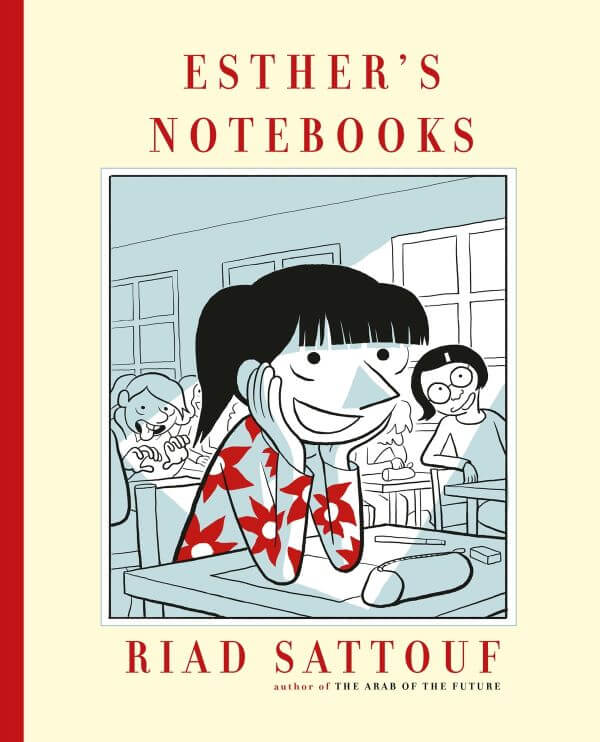This is an image of the cover of a book titled "Esther's Notebooks" by Riyad Satouf, the author of "The Arab of the Future." The cover features a pale yellow background with a bold red frame and binding on the left. The title "Esther's Notebooks" is prominently displayed at the top in red, all capital serif letters. The center of the cover depicts a young girl, animated and smiling, with her hands resting on her cheeks. She wears a white and red shirt with red flower-like patterns and has a short ponytail. The girl appears attentive, perhaps in a classroom setting, drawing attention to her eagerness. In the background, other children are visible, with one boy seemingly making fun of her, adding a layer of narrative to the illustration.